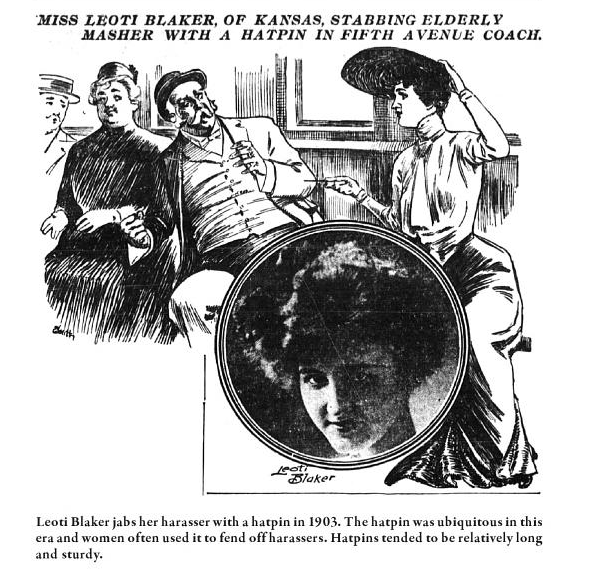This detailed black and white hand-drawn image, resembling a vintage newspaper depiction, portrays an event on a 5th Avenue Coach where Miss Leoty Blaker of Kansas is depicted defending herself from an elderly masher by stabbing him with a hat pin. In the vertical drawing, several individuals, including mustached men in suits and hats, are seen seated across from a resolute Miss Blaker, who is wearing a large hat and a gown. Holding her hat with one hand, she thrusts a long and sturdy hat pin towards the man's arm, conveying a sense of urgency and fear as he recoils. The background suggests a train coach setting with visible windows and walls. Above and below the illustration, text captions detail the incident, mentioning the ubiquity of hat pins in 1903 as a common tool for women to fend off harassers. Additionally, the image includes a circular close-up of Miss Blaker's face, emphasizing her determined expression and framing the narrative of her bold self-defense.